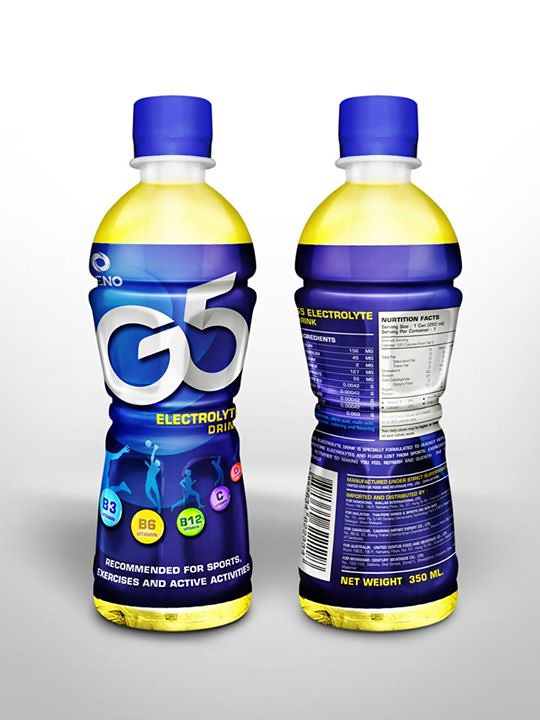This promotional image features a likely artistic render or computer-generated mock-up of an electrolyte drink called G5. Set against a background that transitions from light gray at the bottom to nearly white at the top, the image prominently displays two bottles side by side to showcase both the front and back labels. The bottle has a blue cap and a clear body filled with a bright yellow liquid, similar in hue to Mountain Dew. 

The blue label on the bottle bears the brand name ENO in small white print at the upper left-hand corner. Beneath it, "G5 Electrolyte Drink" is written in larger letters. Surrounding the text are colorful bubbles in blue, yellow, green, pink, and purple, indicating the presence of vitamins B3, B6, B12, C, and D. The label also states that the drink is recommended for sports, exercises, and active activities, and features images of people engaging in activities like volleyball, running, and golfing. 

On the back label, though the small print is unreadable, it includes a nutritional information section and lists the net weight as 350 milliliters, suggesting it might be a non-American product given the metric measurement.